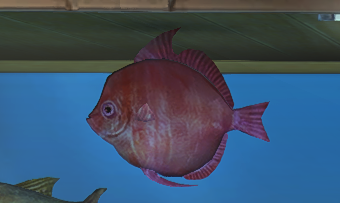The landscape-oriented photograph presents a vivid depiction of a fish tank scene. Dominating the center is a striking, flat red circular fish, distinguishable by its unusual pink eye and a series of fins: one at the top, one at the bottom, a tail fin, and small swimming fins along its side. The fish’s round, wide body features a distinctive long fin that extends from its forehead to its tail. The background is a blend of bright blue water occupying the lower half and a brownish-green upper section, possibly suggesting the top of the tank or a nearby dock. In the lower left corner, partially visible, is another fish, primarily green with a top fin and a crescent-shaped tail fin. The overall atmosphere gives a slightly surreal impression, likening it to a scene from a video game rather than a real-life fish tank.